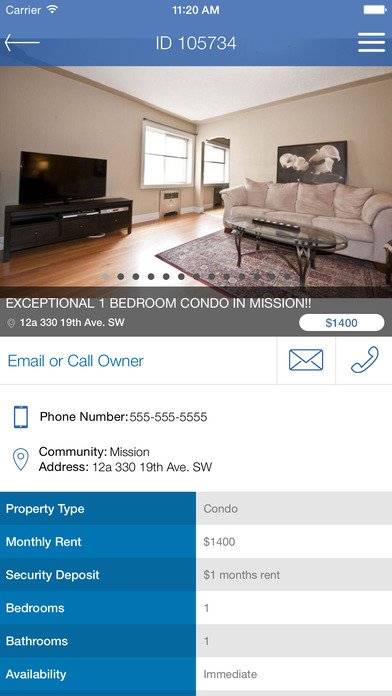This is a screenshot of a mobile app for property finding. The top section features a blue background with a property ID and number prominently displayed. Below this, there is a large, high-resolution photo showcasing the interior of an apartment. Directly under the photo, bold white text reads "Exceptional One-Bedroom Condo in Mission."

On the bottom left corner of the photo, there's a location icon followed by an address in small white letters. The bottom right corner has a white bubble containing the price, "$1,400," in large blue numbers. Beneath the photo, there are large blue letters prompting users to "Email or Call Owner," accompanied by an envelope and a telephone icon.

Further down, the screen is divided into two columns. The left column, highlighted in blue, lists categories such as property type, monthly rent, security deposit, bedrooms, bathrooms, and availability. The right column, in gray and white, provides the corresponding details: the property type is "Condo," the monthly rent is "$1,400," the security deposit is one month's rent, there is one bedroom, one bathroom, and the availability is "Immediate."

Additional contact information is provided in the middle of the screen, with a phone icon to the left followed by a phone number, and a location icon to the left followed by the community and address.